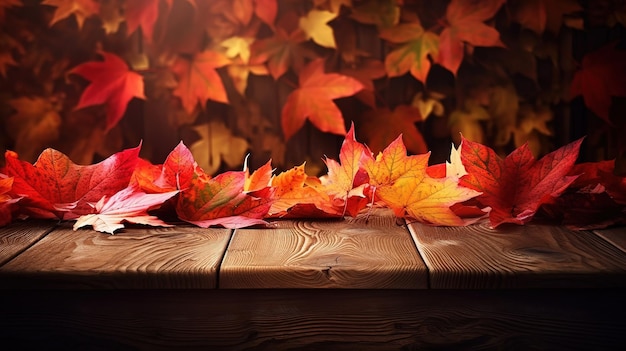This image is a highly detailed, well-lit photograph, potentially digitally captured, showcasing an autumnal scene. The foreground features the edge of a prominent, grainy wooden desk or table, bathed in studio-like lighting that accentuates its dark tones and textures. Atop this wood surface, a collection of vibrant, fall-colored maple leaves in shades of red, orange, and yellow are arranged. The leaves' warm hues are beautifully highlighted by the overhead lighting, casting defined shadows underneath.

In the background, there is an out-of-focus vertical expanse adorned with similarly colored maple leaves, creating a layered effect. The vertical background gives the impression of a wall or hanging surface, adding depth and a sense of enclosure to the scene. The entire composition appears meticulously staged, with both the foreground and background leaves contributing to a cohesive and immersive autumnal atmosphere.